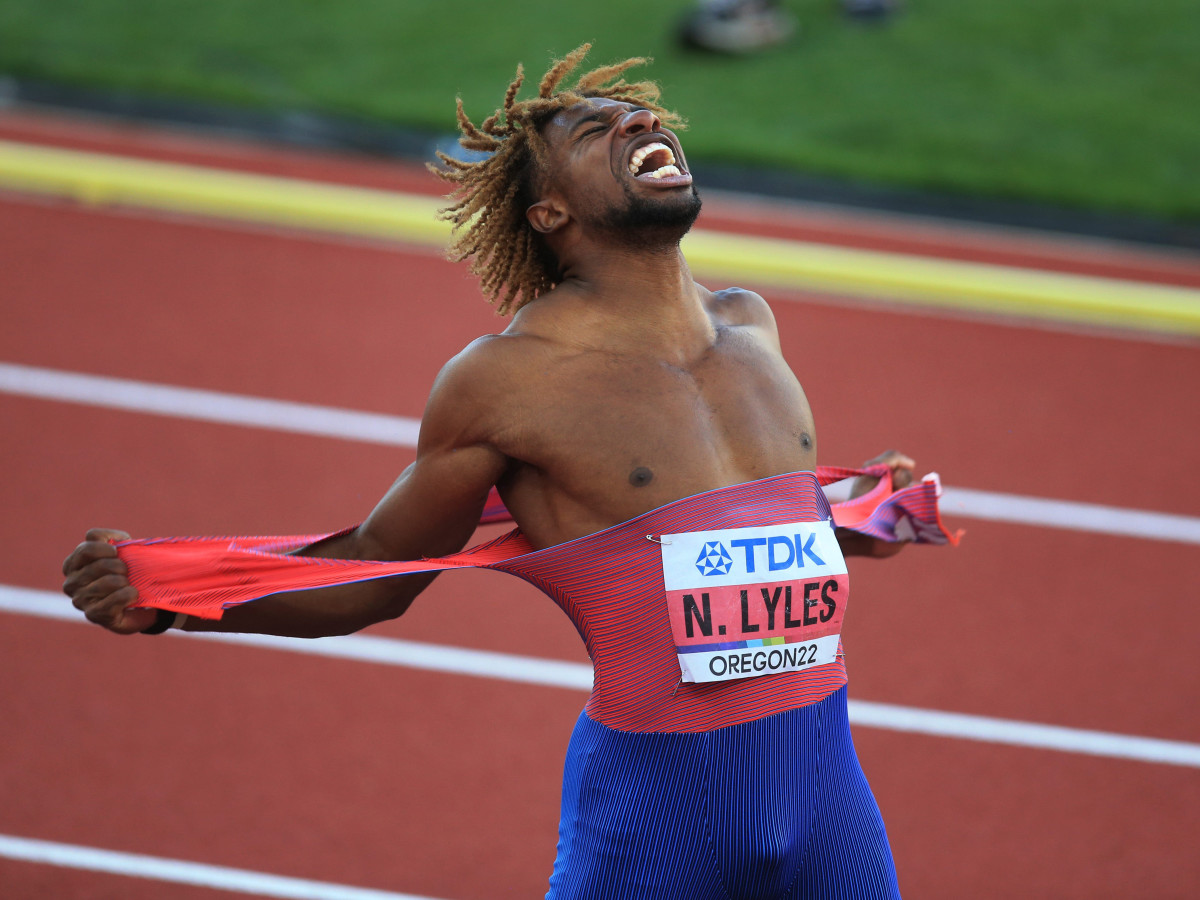In this dynamic and emotional photograph, a black male runner is captured at a triumphant or intensely emotional moment during a race. The runner, N. Lyles, is prominently featured in the center of the landscape-oriented image, exuding a powerful sense of achievement or relief. His head is thrown back with his eyes closed and mouth wide open, possibly screaming in ecstasy or agony. His long braids are caught in mid-motion, flying around his head, adding to the sense of energy and movement.

He is in the process of tearing off his tight red tank top, revealing a muscular, lean physique. The tank top carries the logo "TDK" prominently on the front, with his name "N. Lyles" underneath in black letters on a red stripe, followed by "Oregon 22." This indicates that TDK is likely the sponsor and that the setting is a competition held in Oregon in 2022.

He wears tight blue shorts that end above the thigh, consistent with typical track and field apparel. The background features a red track with white lane markings and a yellow line at the track's edge, beyond which lies a blurry patch of green grass, indicating the infield area of a track and field venue. The overall imagery strongly conveys the intensity and passion of competitive racing.